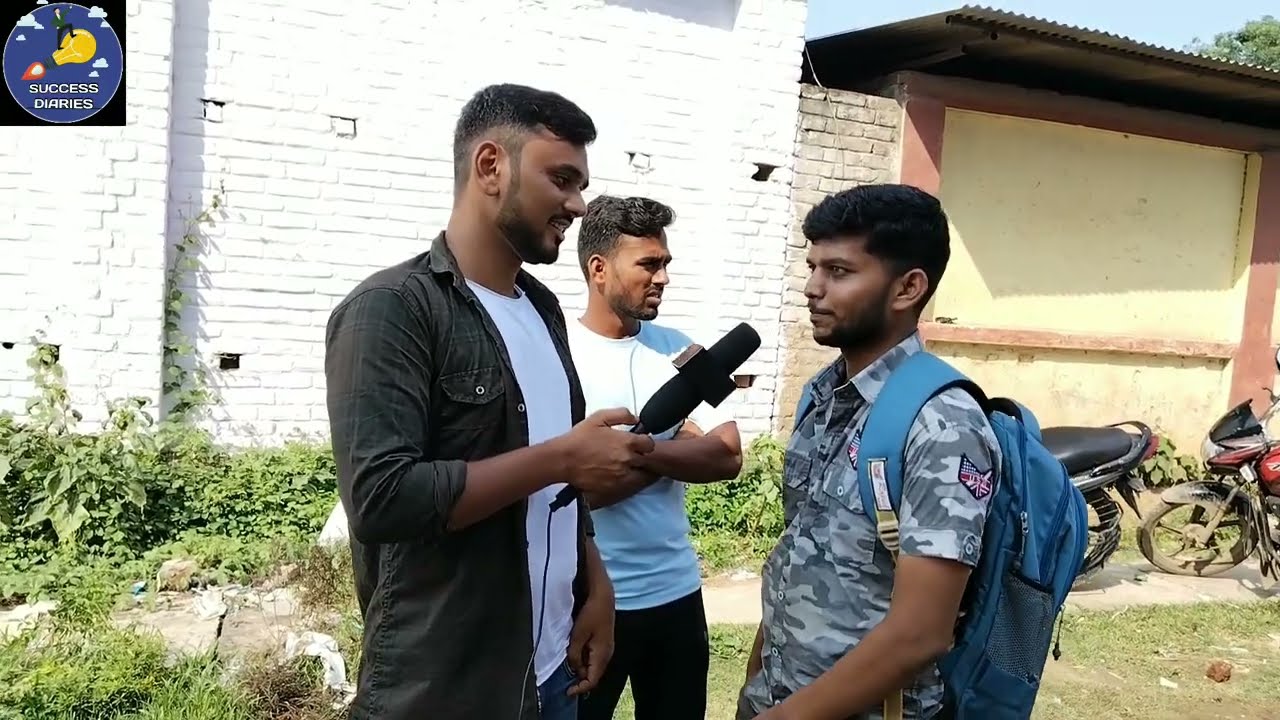The image portrays three young men, likely in their early to mid-twenties, standing outside on a grassy, weedy area. They all have darker skin tones and short black hair. The man on the right, who appears to be the main focus, is being interviewed; he is wearing a light gray camouflage short-sleeved shirt and a light blue backpack. He's holding a black microphone extended by the man on the left, who is dressed in an unbuttoned dark brown jacket with a white t-shirt underneath. This interviewer has short black hair, shaved on the sides, and a thin beard. The third man stands in the center background, wearing a simple white t-shirt and dark pants, looking off to the right. Behind the group is a white brick wall transitioning to a beige wall with red wood accents. In the lower right corner, two motorcycles are visible, adding to the outdoor setting. The background also includes a "Success Diaries" logo with a symbol resembling a microphone or light bulb in yellow, blue, and pink, and a clear blue sky can be seen above the top of a tree.